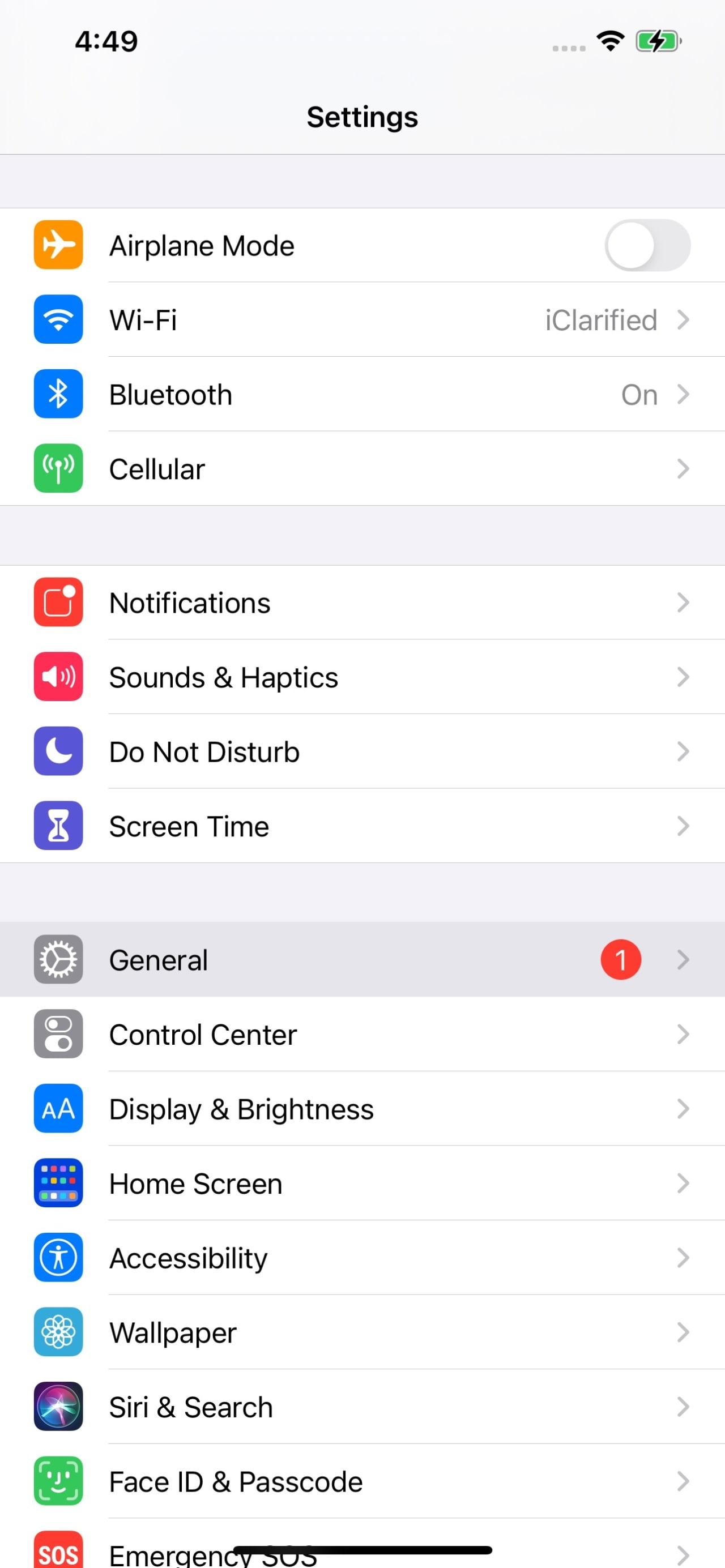The image depicts the "Settings" screen of a smartphone, showcasing various system preferences and statuses. At the top of the screen, the time reads 4:49, and icons indicate that the device is connected to data or Wi-Fi. The battery indicator, colored green, signifies that the battery is currently charging.

Below the header, the word "Settings" is prominently displayed. The settings options are listed in the following order:

1. **Airplane Mode**: Disabled
2. **Wi-Fi**: The current status is shown in gray with an information symbol and an arrow pointing to the right.
3. **Bluetooth**: Enabled, with an accompanying status displayed.
4. **Cellular**: Includes an arrow indicating further options.
5. **Notifications**
6. **Sound & Haptics**
7. **Do Not Disturb**
8. **Screen Time**
9. **General**: Marked by a red circle with a '1' inside it, indicating a pending update or notification.
10. **Control Center**
11. **Display & Brightness**
12. **Home Screen**
13. **Accessibility**
14. **Wallpaper**
15. **Siri & Search**
16. **Face ID & Passcode**
17. **Emergency SOS**

Each option on the list features a corresponding icon, which presents a range of colors such as orange, blue, green, red, purple, and black. All options, except for "Airplane Mode" and "Bluetooth," also have an arrow pointing to the right, suggesting further configurable settings. 

Overall, the screen is structured in a clear, intuitive layout, allowing easy navigation through the various settings.